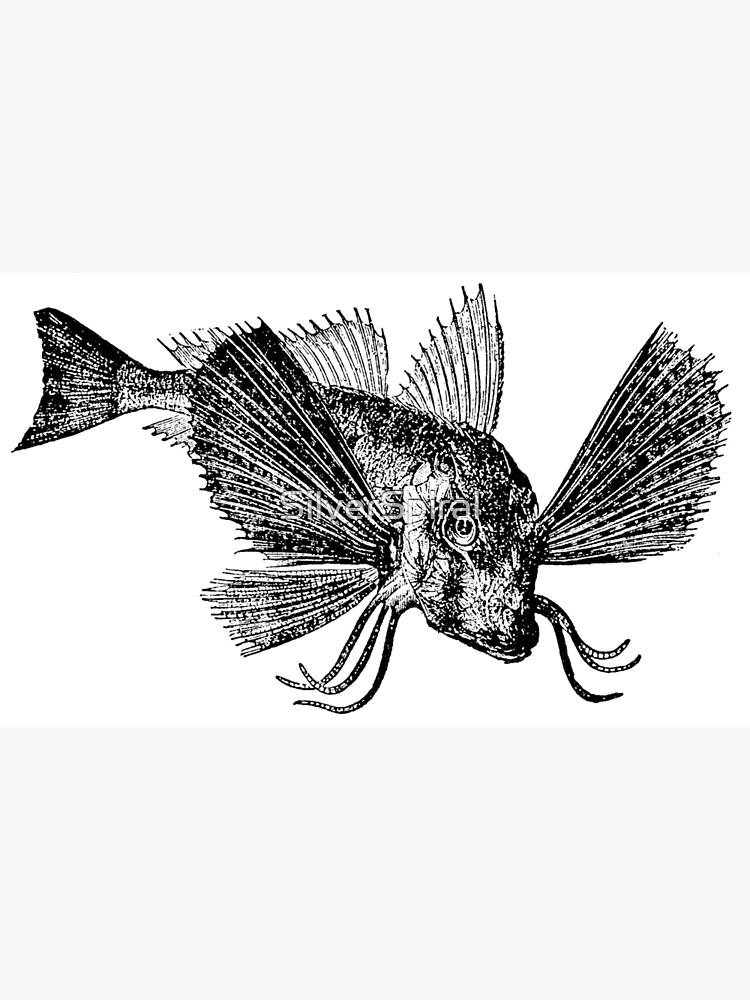The image showcases a detailed, black and white hand-drawn fish, framed by gray bars that letterbox the top and bottom 25-30% of the image. The fish, likely a catfish, is oriented towards the five o'clock direction, with a slightly curving body to the right. Its face is somewhat flat with a protruding mouth, and it features six long, tentacle-like whiskers (three on each side) under its jaw. The fish’s fins are meticulously detailed, with fan-like, needle-textured pectoral fins extending from its cheeks, and three dorsal fins along its back as well as a fin on its underbelly. The drawing also highlights a large caudal fin at the tail's end, contributing to its overall intricate and lifelike appearance.